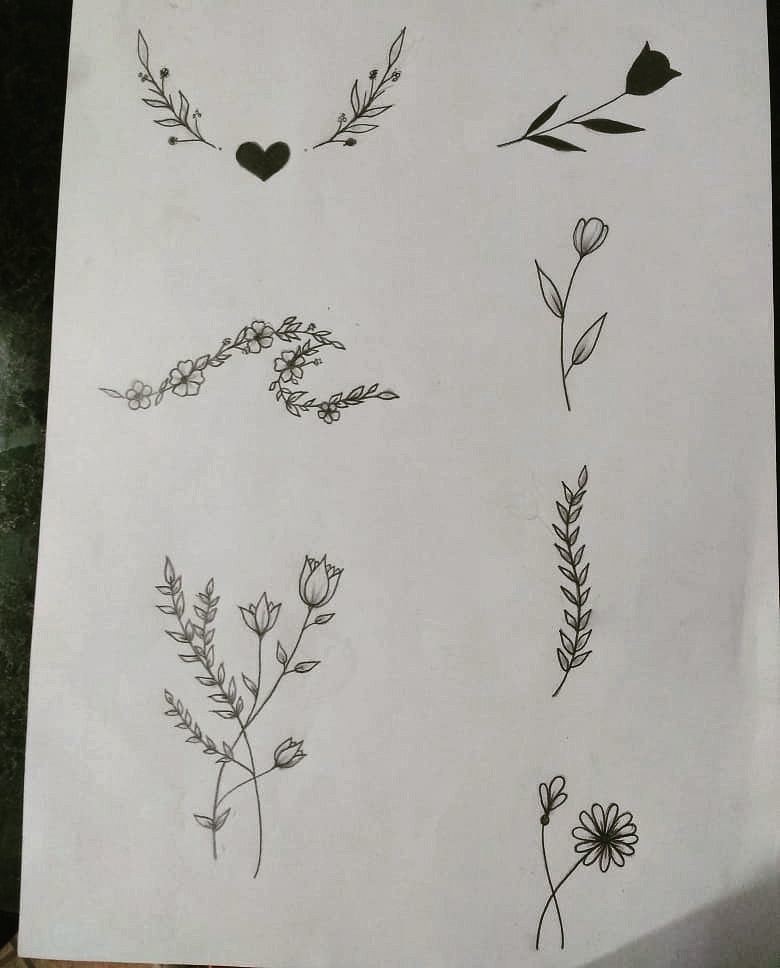A collection of intricate pen drawings on paper, showcasing the remarkable skill of the artist. The illustrations appear to be freehand, executed without the aid of stencils or reference points, highlighting the artist's expertise. In the bottom left corner, delicate flowers intertwine with branches to form an 'X' shape. Central to the composition is a branch with flowers, gracefully curving to resemble a wave. To the right, a single tulip stands vertically, contrasting with another tulip above it, which is fully shaded in black, suggesting the silhouette of a tulip leaning to the right. Adjacent to this, a heart emerges, adding a sentimental touch to the artwork.